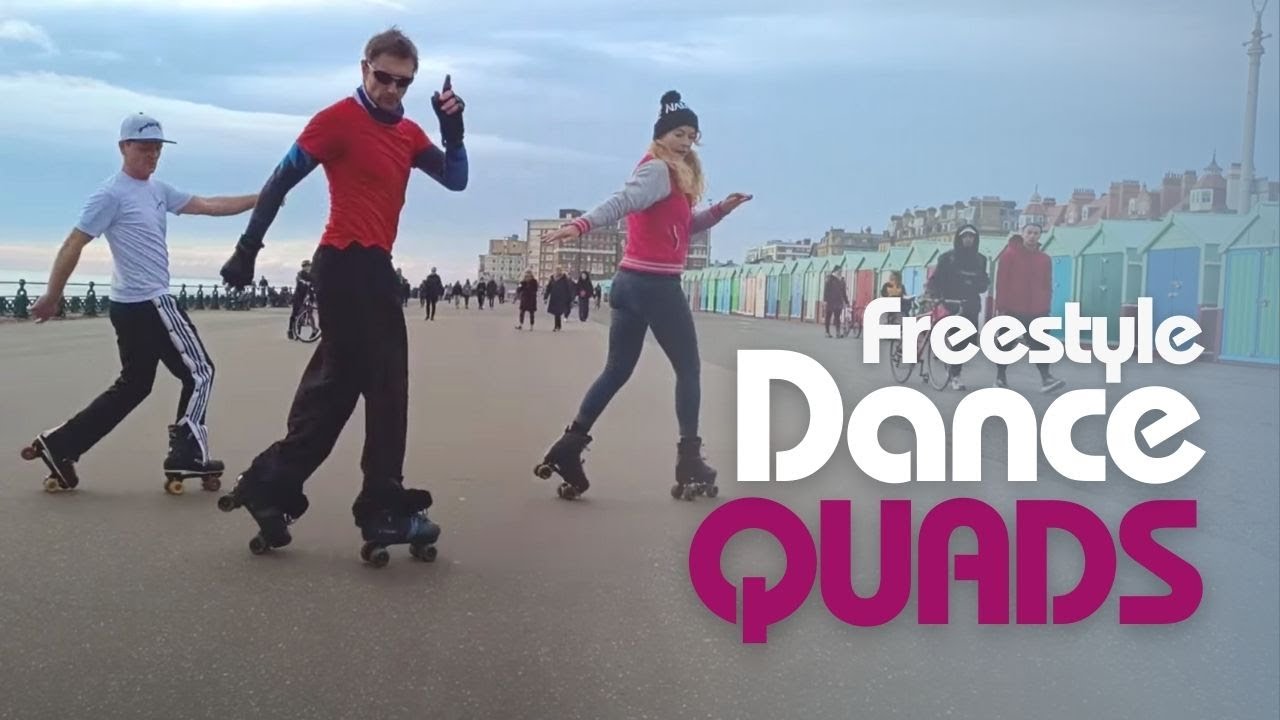The image depicts an outdoor beachside scene under a light blue sky, with a view of the ocean in the background to the left. In the middle of the picture, three dancers—two men and one woman—are performing synchronized moves on roller skates, specifically four-wheeled quads. The first man, on the left, wears black pants with white stripes and a white shirt. The second man, positioned centrally, wears black pants paired with a red shirt over a black undershirt. The woman, on the right, sports black pants, a white and pink jacket, and a red beanie. To the right of the image, the words "Freestyle Dance Quads" are visible, with "Freestyle Dance" in white and "Quads" in purple capital letters. The scene is set on a concrete area bordered by multicolored sheds and tall buildings, possibly hotels, which extend into the distance on the right side of the image. A few onlookers can be seen in the background, walking and observing the dancers.